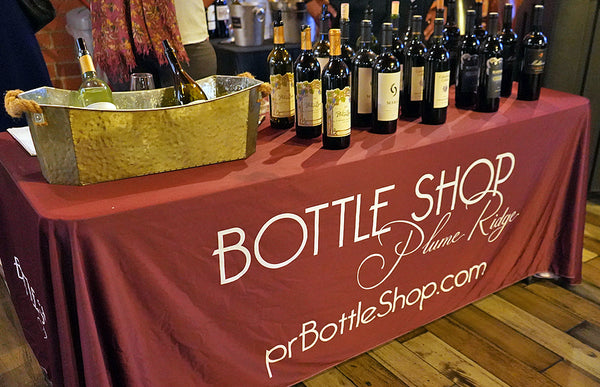This photograph captures a well-arranged display table, presumably in an alcohol or wine store setting. The table, covered in a red tablecloth bearing the text "Bottleshop, Plum Ridge, prbottleshop.com" in white lettering, is set against a background of various brown and beige shades of a wooden floor. The main focus of the image is the assortment of wine bottles organized on the table. There are approximately 15-20 bottles of different types, with some grouped three or four deep. To the left side of the table, a prominent gold ice bucket with rope handles contains two bottles of wine, and beside it sits a wine glass. In the background, there appears to be another table with a similar silver metallic bucket, contributing to the overall ambiance of a wine-tasting or promotional event. Though slightly obscured, there might be a person nearby, potentially wearing brown pants, a white shirt, and a long red scarf, adding a touch of human presence to the scene.